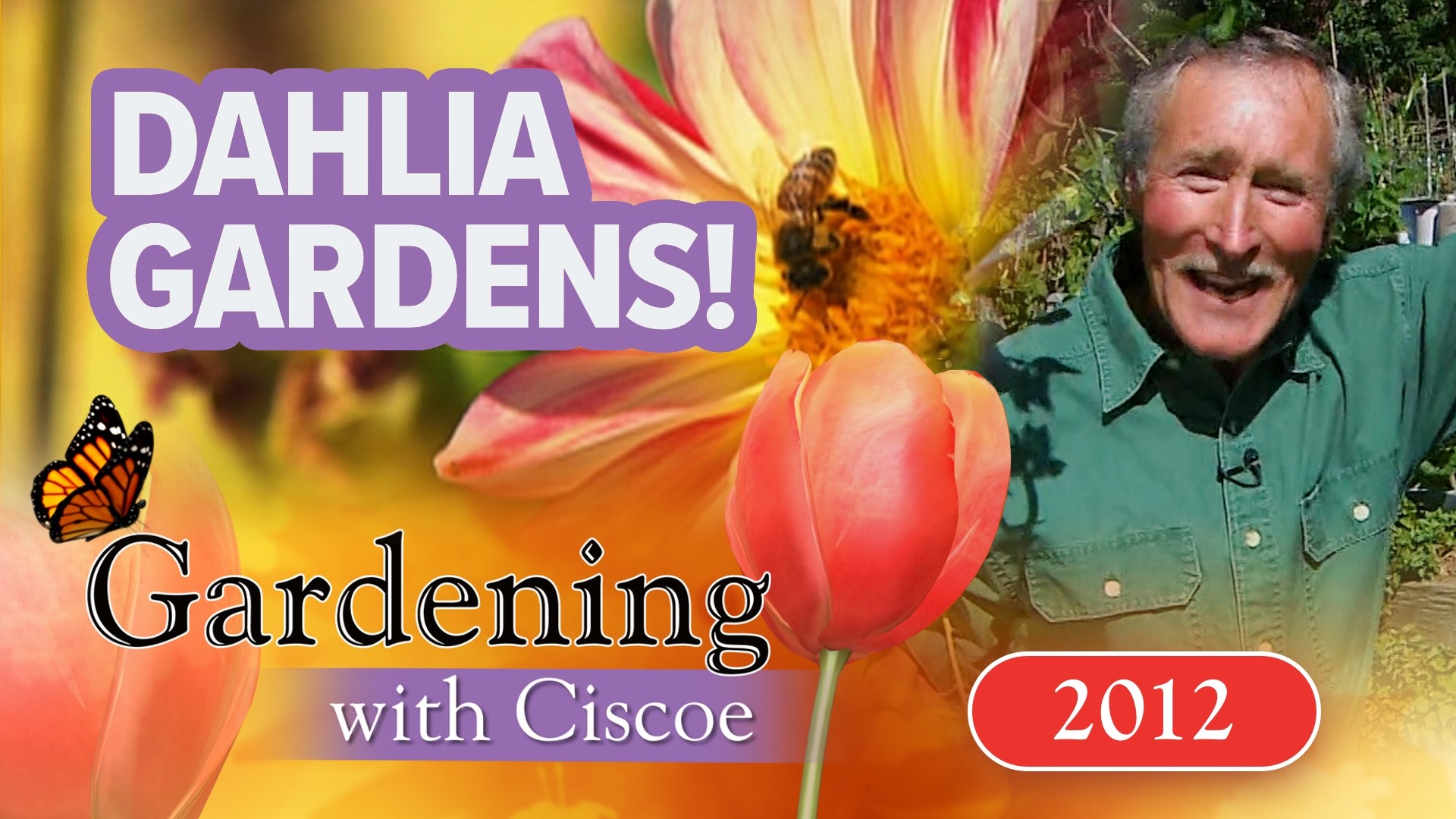The image is a landscape-oriented advertisement, possibly a thumbnail for a YouTube video or a podcast title image, about "Gardening with Cisco." It prominently features the text "Dahlia Gardens!" in the upper left-hand corner in white capital letters with a medium purple outline. Below this text, in the lower left-hand corner, the words "gardening with Cisco" appear in black and purple/white text, respectively, accompanied by an orange and black butterfly perched on the "G" of "gardening." The lower right-hand corner features the year "2012" on a red background with white text. On the right half of the image is a close-up of an older man, presumably Cisco, who has salt-and-pepper hair and mustache, and is clad in a green long-sleeve collared shirt with two front pockets and white buttons. The left side of the image showcases vibrant flowers, including red, yellow, and orange hues, with bees visible on some of the blossoms.